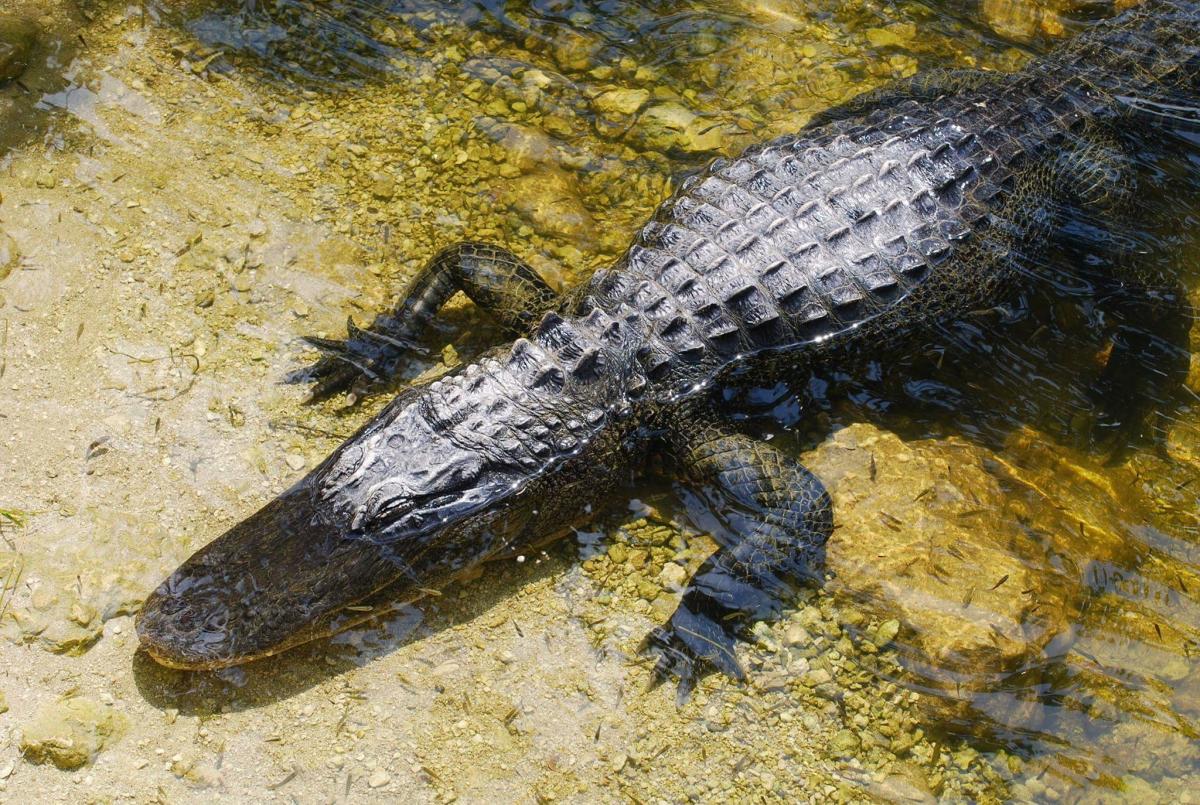In this rectangular photograph taken from above, we see a crocodile submerged in a shallow, clear body of water, revealing intricate details of its environment and physique. The water's transparency allows us to observe a yellowish floor interspersed with variously colored stones—white, light brown, and black—and ropes. The crocodile, mostly submerged except for parts of its scaly, dark-gray to black body, stretches diagonally with its head in the lower left corner and its partially hidden tail towards the upper right. The head features a triangular shape that rounds at the snout, and its four legs, splayed out with visible black claws, contribute to its menacing presence. Small fish swim around the crocodile, adding life to the serene scene. The scales run in ridges from its head down its leathery back to the tail, creating a visually textured pattern. The photograph captures an intricate moment, showcasing the stillness of the reptile, possibly waiting to snap at an unsuspecting fish.